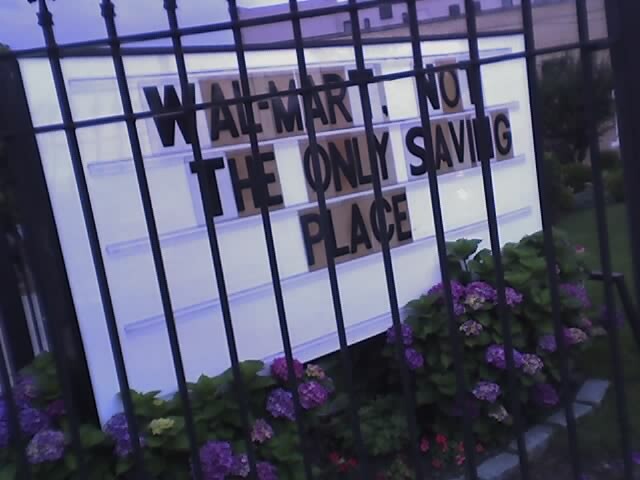This color photograph captures an outdoor church sign, cleverly aimed at attracting attention with humor. The sign, with a black border and white background, displays the message in black letters: "Walmart, not the only saving place." This playful pun suggests the church is an inviting, fun community. The sign is partially hidden behind a wrought iron black metal fence featuring vertical and horizontal railings. In front of the sign and beneath the fence, vibrant purple flowers bloom amidst lush green foliage and bushes, adding a touch of natural beauty. To the right of the sign, the edge of the church building is visible. The sign appears to have a strip light for potential illumination, though it is not lit in the photograph. The sky or possibly a wall in a medium dark blue shade can be seen above the sign, and grass surrounds the base of the wrought iron fencing. The sign itself is positioned on a slight diagonal, with the left side closer to the edge of the frame.